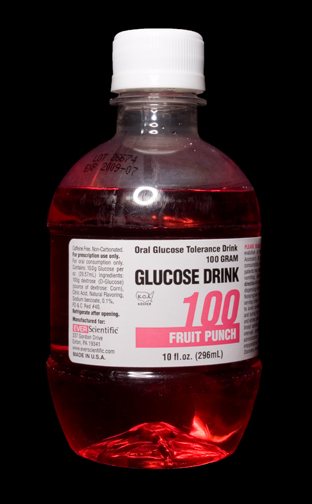The image depicts a small bottle set against a completely black background. The diminutive bottle is labeled "Glucose Drink 100" and contains a fruit punch-flavored liquid. The bottle holds 10 fluid ounces (296 milliliters) of this beverage, designed for oral glucose tolerance tests, and contains 100 grams of glucose. The bottle is capped with a white lid and features a white rectangular label on one side. The label includes black text, with "Fruit Punch" highlighted in white against a pink background. Due to the image clarity or size, the expiration date and smaller text containing warnings and directions are illegible. The bottle itself is enclosed in a transparent plastic and contains a red liquid, reflecting its fruit punch flavor.